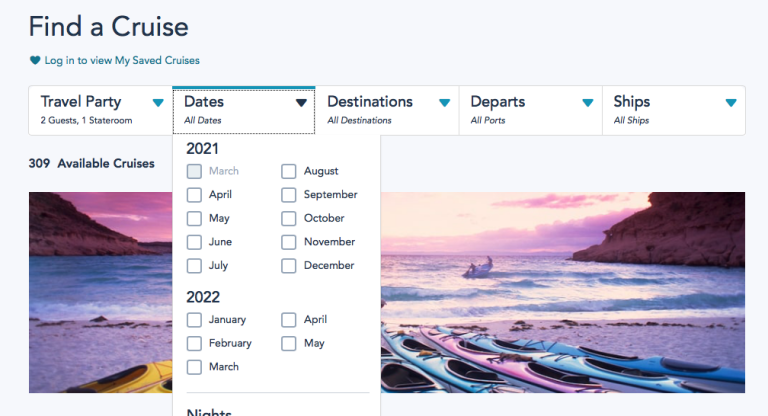The image features a user interface with a gray background. At the top, there's a heading in bold text that reads "Find a Cruise." Below this, a blue heart icon accompanies the text "Log in to view my saved cruises." Further down, there's a selection box labeled "Travel Party," displaying "two guests, one stateroom." Adjacent to this, another box allows users to select "Dates," currently set to "All Dates." A drop-down menu provides monthly options spanning from March to December 2021 and January to May 2022.

To the right, filtering options are available with headings such as "Destinations" (set to "All Destinations"), "Departs" (set to "All Ports"), and "Ships" (set to "All Ships"). The lower portion of the interface showcases a picturesque beach scene. The beach is framed by mountains on both the left and right, beneath a sky tinged with a purplish hue. The sandy shore is dotted with an array of kayaks in vibrant colors—yellow, purple, and blue—neatly arranged on the sand.